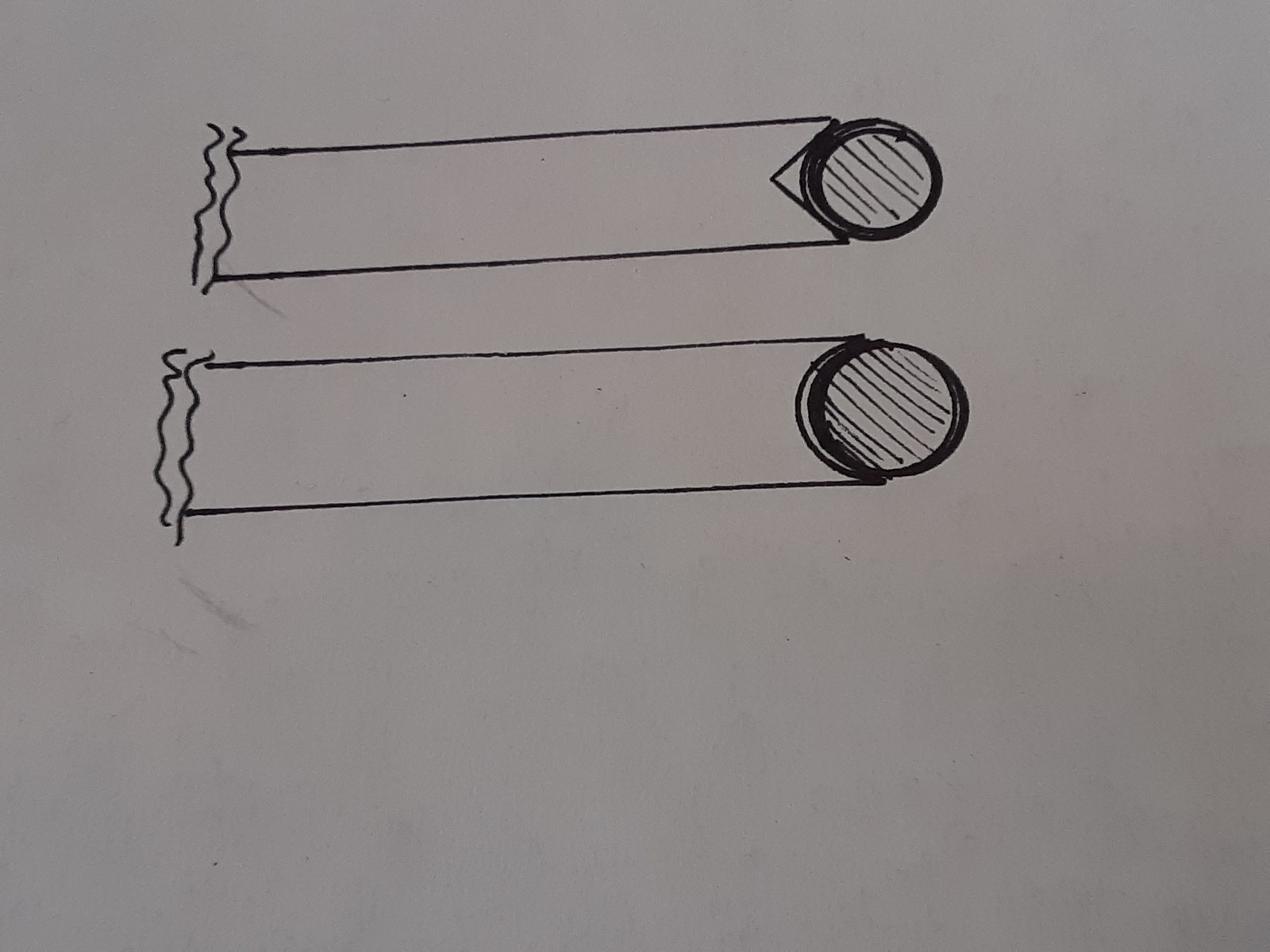This detailed pen and ink drawing showcases two elongated, rectangular objects positioned vertically, one above the other, on a crisp sheet of off-white paper. Each object features wavy lines running horizontally across the left side, adding a textured element to the otherwise linear design. Both rectangles terminate at the right end with a prominent circular shape, characterized by a bold circumference and intersected by diagonal black lines. The circular element serves as a focal point, differing slightly in its attachment to each rectangle: the top rectangle has a triangle-shaped notch supporting the circle, while the bottom rectangle exhibits a smooth, curved indentation housing the circular form. The intricate details and precise arrangement of these geometric shapes highlight the meticulous craftsmanship involved in this artwork.